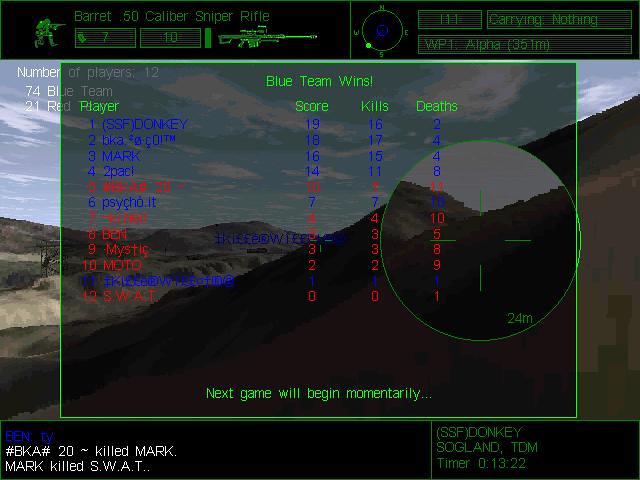In this detailed video game screenshot, the viewer's attention is first drawn to the top-left corner where an emblem depicting a sideways person with a green gun is visible. Below this, the text reads "Barrett .50 Cal Sniper Rifle" accompanied by an icon of a sniper rifle, also in green. Next to this, there is a green rectangle featuring the number "7" with gray shading, and to its right, another green rectangle with the number "10".

On the right-hand side of the screen, a compass displaying the directions N-E-S-W is prominently shown. Adjacent to the compass are a series of rectangular shapes containing various words. Beneath this interface element lies the gameplay screen, which showcases a rugged and rocky mountainside landscape.

In the lower right corner, a target reticle is visible, designed as a green circle with four green lines extending outward. Accompanying this, a series of letters arranged in a pattern reads: "blue, blue, blue, blue, red, blue, red, red, red, red, blue, red." This is indicative of the divided teams, along with their respective scores, kills, and deaths.

Central to the screen, in bold green text, the message "Blue team wins" is displayed, followed by "Next game will begin momentarily". The entire message is encased within an outer green frame. Below this, the screen transitions to a black background filled with additional textual information.